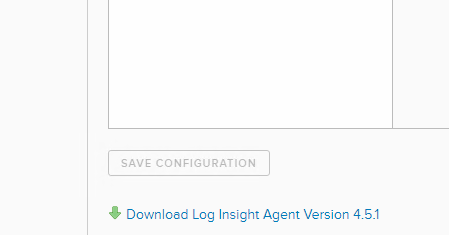This image displays a focused view of a page highlighting a partially obstructed white chart or box at the top. Directly below this box, there is a clearly visible "Save Configuration" button. Underneath this button, a prominent blue link reads "Download Log Insight Agent Version 4.5.1," with the text styled so that the first letter of each word is capitalized, while the remaining letters are in lowercase. Accompanying this link, there is a green arrow pointing downwards on its left side. The rest of the page appears blank, further accentuating the outlined sections and the elements within them.